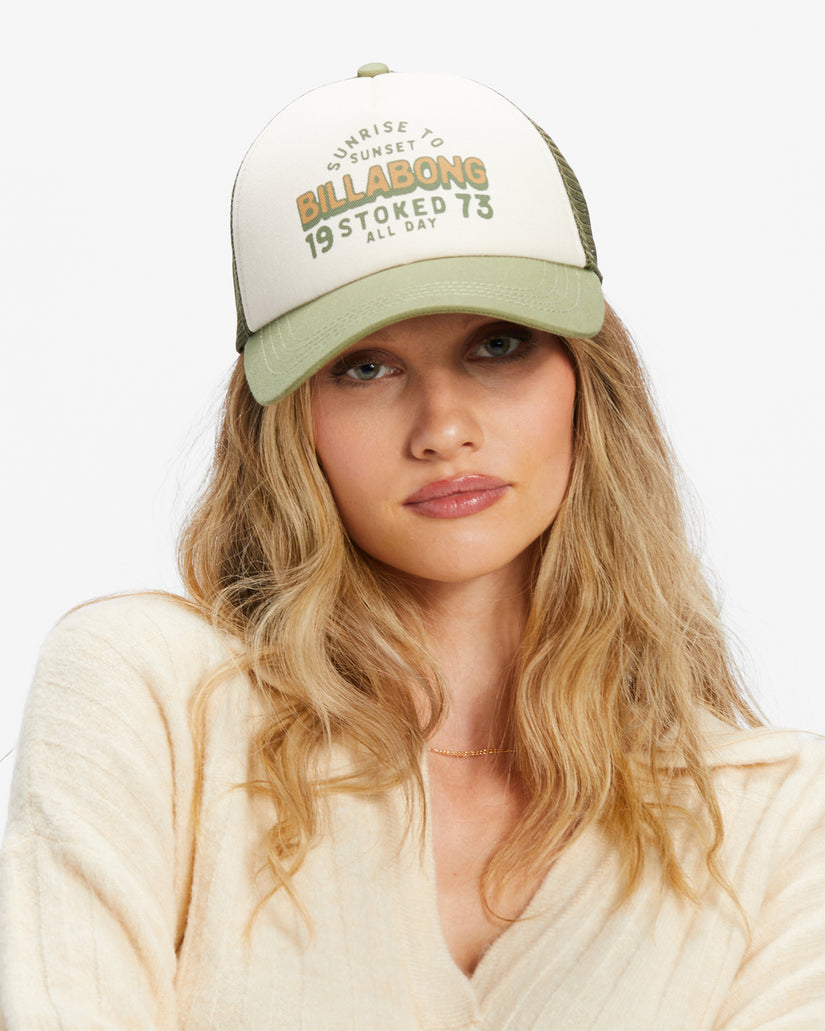This photograph captures a close-up of a young model from the chest up against a stark white background. She is wearing a white, V-neck sweater accessorized with a delicate gold chain necklace. Her shoulder-length blonde hair frames her face, accentuating her tan complexion and subtly enhancing her pink-rose lipstick. The most prominent feature is her trucker-style hat, designed with a green visor and an olive mesh back. The front of the hat is white with a mix of gray-green and yellow lettering that reads, "Sunrise to Sunset, Billabong, 19 stoked, 73 all day." Billabong is highlighted in yellow with a shadow effect. The woman’s blue eyes, serious expression, and slightly tilted head suggest she is modeling the hat, making it the focal point of the image.